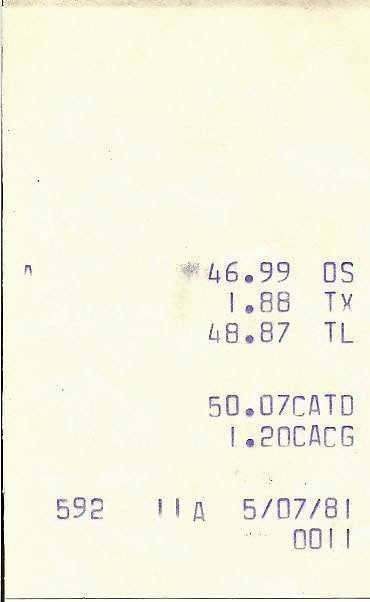This image showcases a close-up view of a receipt printed on white paper. The receipt contains several lines of text and numbers:

1. The first line displays "46.99 OS".
2. The second line shows "1.88 TX".
3. The third line reads "48.87 TL".
4. After a small gap, the fourth line states "50.07 CATD".
5. The fifth line mentions "1.20 CACG".
6. Following another gap, the final line is aligned close to the edge of the receipt with no indentations. It reads "592, II, 5/07/81". The last row contains the numbers "0011".